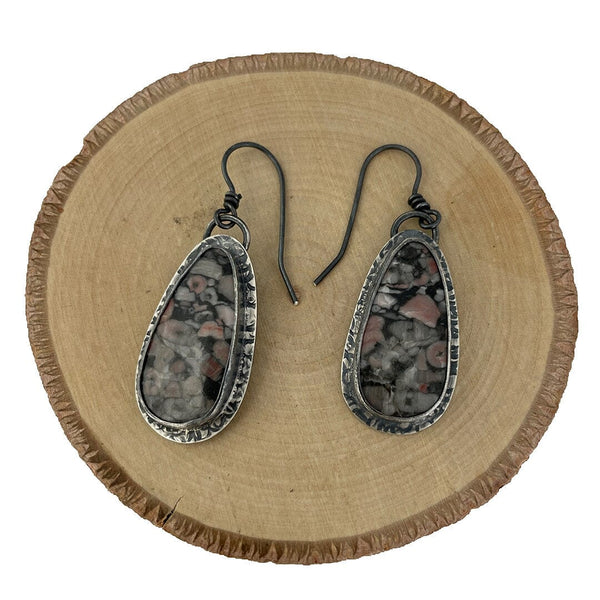The image shows a pair of large, teardrop-shaped decorations that resemble earrings, laying on a circular, artificial tree stump. The stump, which has a soft brown interior with concentric wood rings and a dark brown rim, provides a striking contrast to the decorations. Each decoration features a metal, egg-shaped case with a stone rim, containing several different types of stones or pebbles compressed together. These decorations have metal hooks at the top, possibly indicating they could be hung or attached elsewhere. The decorations are identical in shape but display slightly different rock patterns in black, gray, and silver tones. The image's plain white background further highlights the intricate details of the wood rings and the unique ornaments.